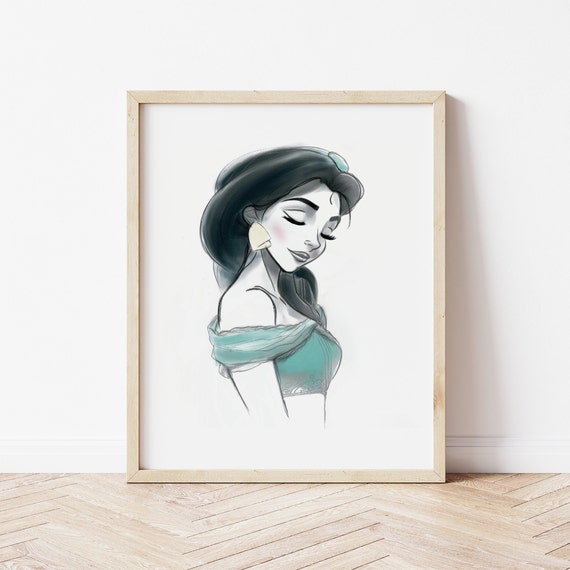A large painting leans neatly against a white wall, resting on a light brown, chevron-patterned wooden floor. The artwork, framed in a thin, unpainted light wood, stands approximately halfway up the wall. It features a young lady depicted against a white canvas background. She has long, dark hair adorned with a circular greenish jewel, matching her teal or cyan sleeveless halter top. The top is draped lightly over her shoulder, exposing her midriff. The young lady has her head tilted down and eyes closed, seemingly serene or in a state of peaceful slumber. She wears long, prominent earrings, resembling small sails or slightly yellow bells. Her face is delicately made up, with perfectly shaped eyebrows, dark lipstick, long eyelashes, and a hint of blush on her cheek. The detailed portrayal, reminiscent of an animated character like Princess Jasmine from Aladdin, infuses a sense of graceful elegance and calm into the room.